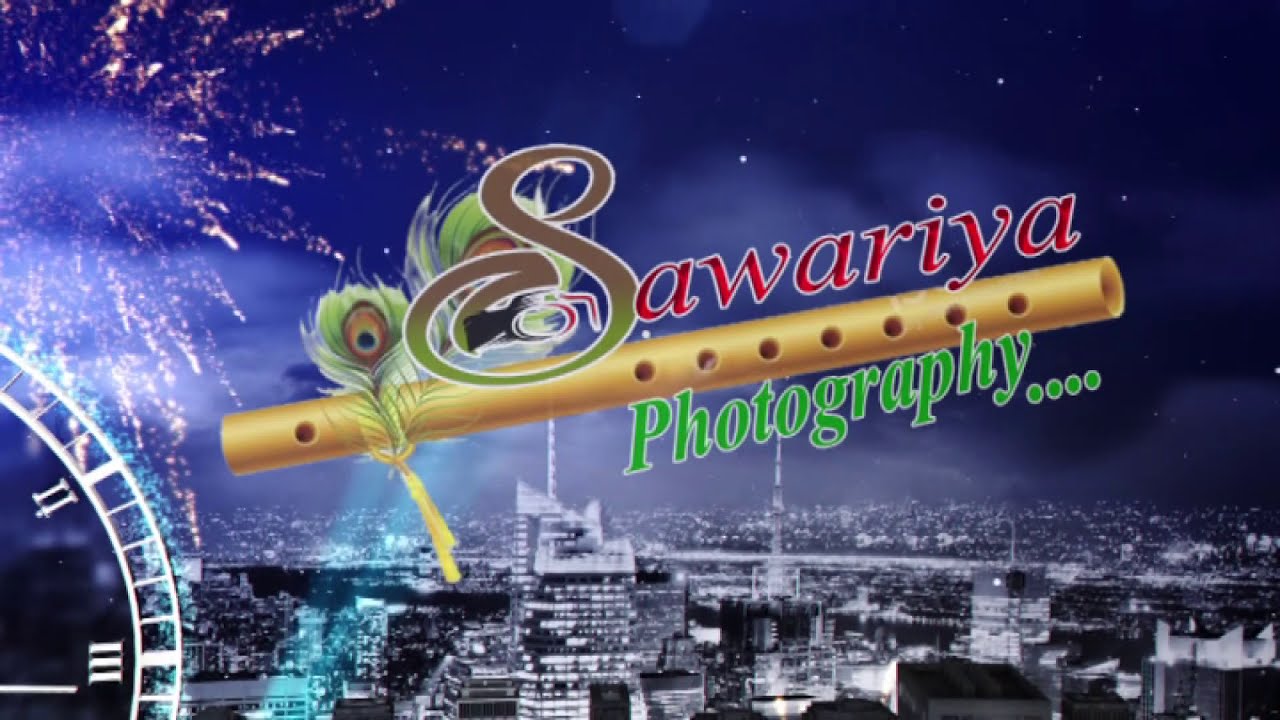The image features a vibrant and intricately designed advertisement set against a bluish-purple nighttime cityscape. The background showcases a detailed black-and-white city skyline with illuminated buildings, antennae, and multiple white stars scattered across the sky. Fireworks explode in the upper left quadrant, adding to the festive atmosphere, while a blue spotlight rises toward the center. In the lower left corner, a partially visible clock displays the numbers 10 and 15.

Prominently overlaid onto the cityscape is a striking graphic design. Dominating the center, a flute-like golden tube with holes runs diagonally across the image. Adorned with a green peacock feather on the left, the design is elegant and eye-catching. To the right of the flute, large and stylized text spells out "SAWARIYA" in a vivid gradient of green and brown for the ornate letter "S," followed by red letters accented with a white outline. Below the flute, the word "PHOTOGRAPHY" is displayed in green text with a white drop shadow, subtly punctuated by four green ellipses. The combined elements create a visually captivating and richly detailed graphic advertisement.